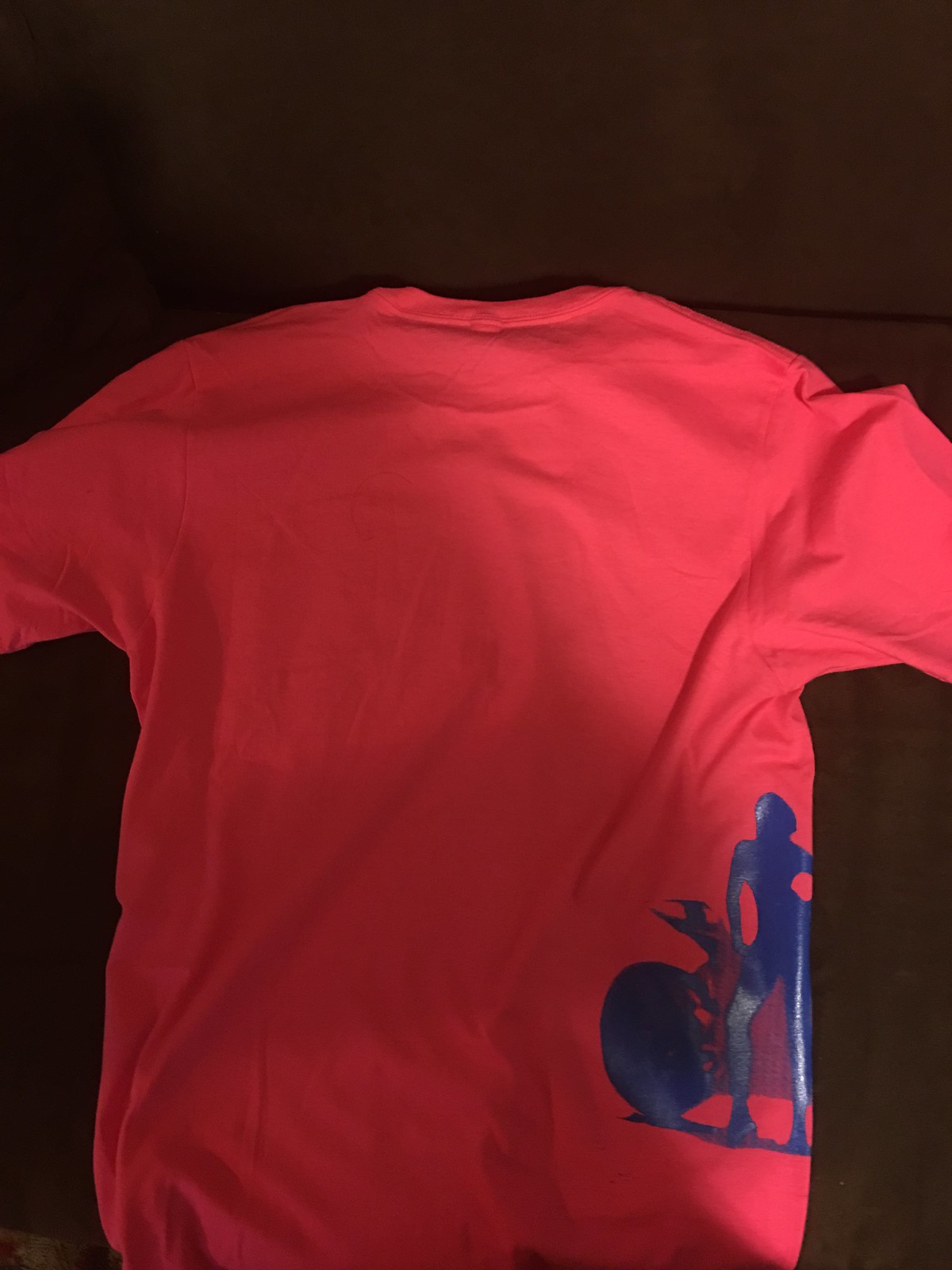The image portrays an orangish-red, possibly salmon-colored short-sleeved t-shirt laid face down on a dark, almost black background. The t-shirt appears wrinkly and not flat, with its back facing the camera. Positioned near the lower right side below the sleeve, there is a blue silk-screened silhouette of a woman. To her left is a round blue object, possibly a ball, with a thin line extending from the object to the under the woman's position. The image features shadows across the shirt, highlighting the creases and folds, with the dark background emphasizing the bright, vivid colors of the t-shirt.